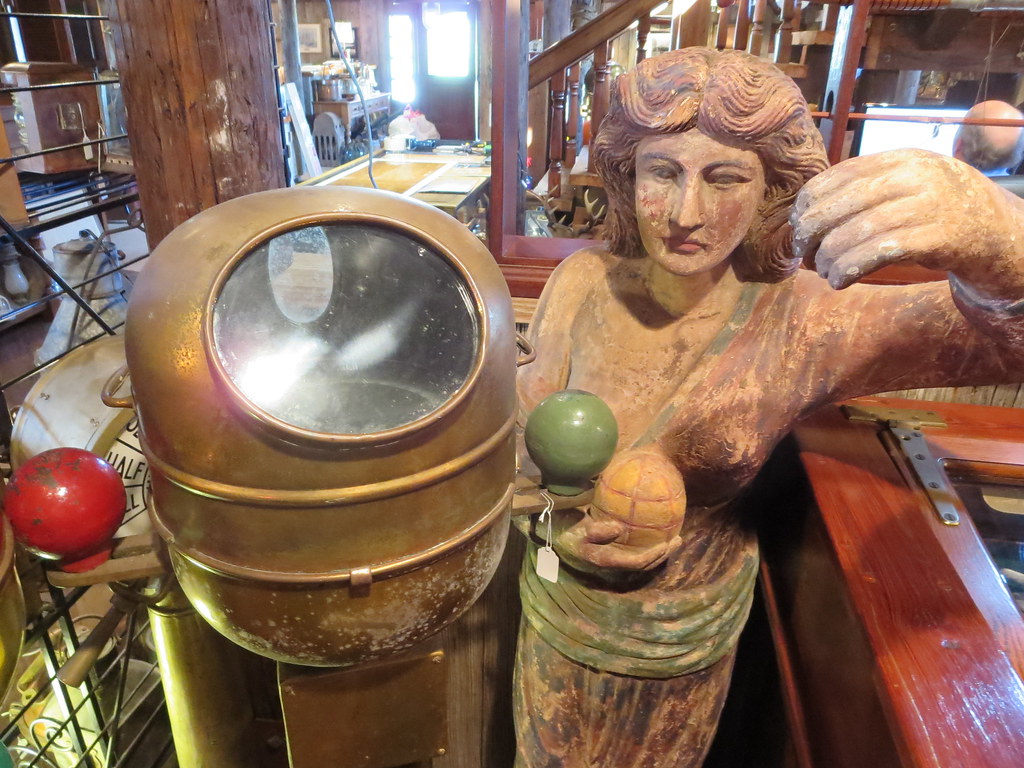In the image, we see an eclectic assortment of objects within what appears to be an antique store. The centerpiece is an intricately carved wooden statue of a woman, slightly off-center to the right. The sculpture features the woman with a subtle smile, detailed hair, and a prominent left arm bent at a 90-degree angle with the hand pointing downward, adorned with a green belt around her waist. She's holding two round balls in her right arm—one green and the other a light orange hue. Adjacent to the statue on its right side is an old bronze metal piece, possibly an antique machine, with a round glass component. In the foreground, an item resembling an astronaut's helmet, potentially a large vase with a wide glass opening, rests near the statue along with a bowling ball placed on a stool.

The background reveals a cluttered yet fascinating scene of various antique items, with a wooden staircase ascending above the sculpture of the woman. Wooden posts and an assortment of eccentric objects with possible price tags suggest this is an antique shop. A messy desk, scattered items on the floor, and a door leading to a window further enhance the chaotic charm of the setting. The color palette is rich with bronze, light yellow, tan, red, green, brown, white, and a touch of gray, adding to the vintage atmosphere of the place.